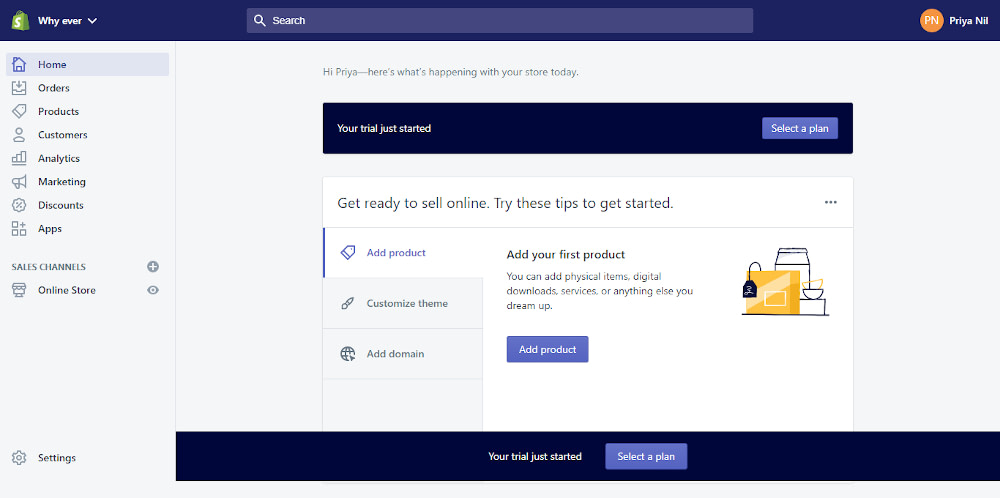The image depicts a website interface designed for buying and selling products. At the top left corner, there is a green paper bag icon with a dollar sign next to it. Directly to the right of this icon, the name "Why Ever" is displayed with a downward arrow beside it. Centrally positioned at the top is a search bar with the word "search" and a white magnifying glass icon inside it. On the top right, the name "Priya Nill" is shown, accompanied by a circle with the initials "PN" to its left.

On the far left side of the image, there is a vertical navigation menu. The menu items listed from top to bottom are: Home (denoted by a home icon), Orders (represented by a download symbol), Products (indicated by a shopping tag icon), Customers (marked by a person icon), Analytics (shown with a graph icon), Marketing (depicted with a blow horn icon), Discounts, and Apps. Below these items is a smaller section labeled "Sales Channels" with the entry "Online Store."

Dominating the central part of the image is a prominent message, "Your trial just started. Select a plan," with the call-to-action "Select a plan" highlighted in white text against a purplish background.